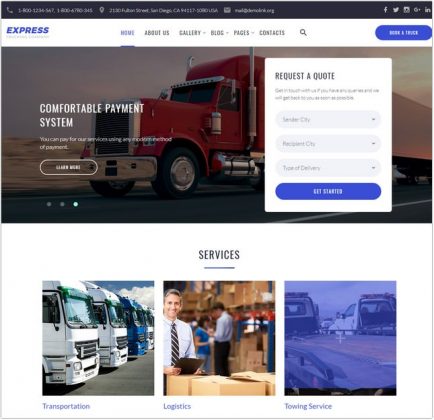At the top of the image, there is a black bar with unspecified text. Toward the right end of this bar, there are five light gray icons in the following order: Facebook, the old Twitter icon, an icon that could be either Instagram or YouTube, Google Plus, and LinkedIn.

Below the black bar, there is a white strip approximately twice the height of the black bar. On the left side of this strip, the word "EXPRESS" is prominently displayed in italicized block letters, colored navy blue. Beneath "EXPRESS," there is smaller text in black or dark gray, which is unreadable.

Centered below this strip is the website's main menu. The menu includes the following tabs: "Home" (selected, underlined, and displayed in dark purple), "About Us," "Gallery" (which has a downward-pointing arrow indicating a drop-down menu), "Blog" (also with a drop-down menu indicator), "Pages" (with a drop-down menu indicator), and "Contacts" (without an arrow, indicating no drop-down menu). Toward the right side of the menu, there is a large blue clickable icon with text in all capitals; although partially unreadable, the last word is "TRUCK."

Below the menu is a large picture banner featuring a semi-truck with a red front and light silver trim. Overlaid on this image is the text "COMFORTABLE PAYMENT SYSTEM" in all capital letters and white font. Additionally, there is smaller illegible text beneath this tagline.